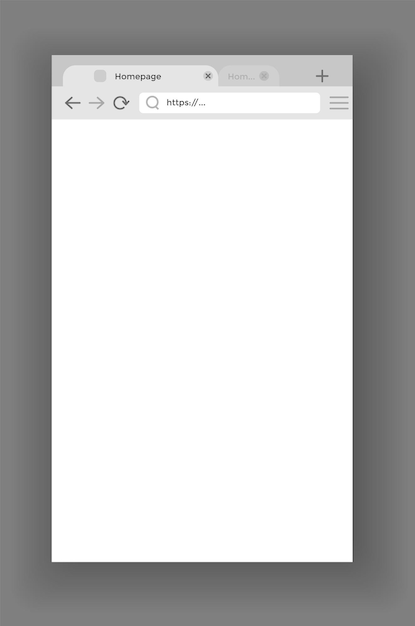The image depicts a slightly faded screenshot of a blank web browser page, which appears to have been captured on a smartphone. The browser displays a single open tab labeled "home page," and the URL bar contains only the initial "HTTPS://...". The entire web page itself is white and devoid of any other images, colors, or text. The screenshot includes familiar browser icons such as back and forward arrows and a refresh button in a light gray area. Surrounding the screenshot is a thick grayish-black border that frames the image and makes it appear somewhat off-center to the left against a black gradient background. A small plus sign is visible in the upper right corner of the browser tab. Overall, the focus is on the stark simplicity and emptiness of the web page, heightened by the subdued and unfocused quality of the screenshot.